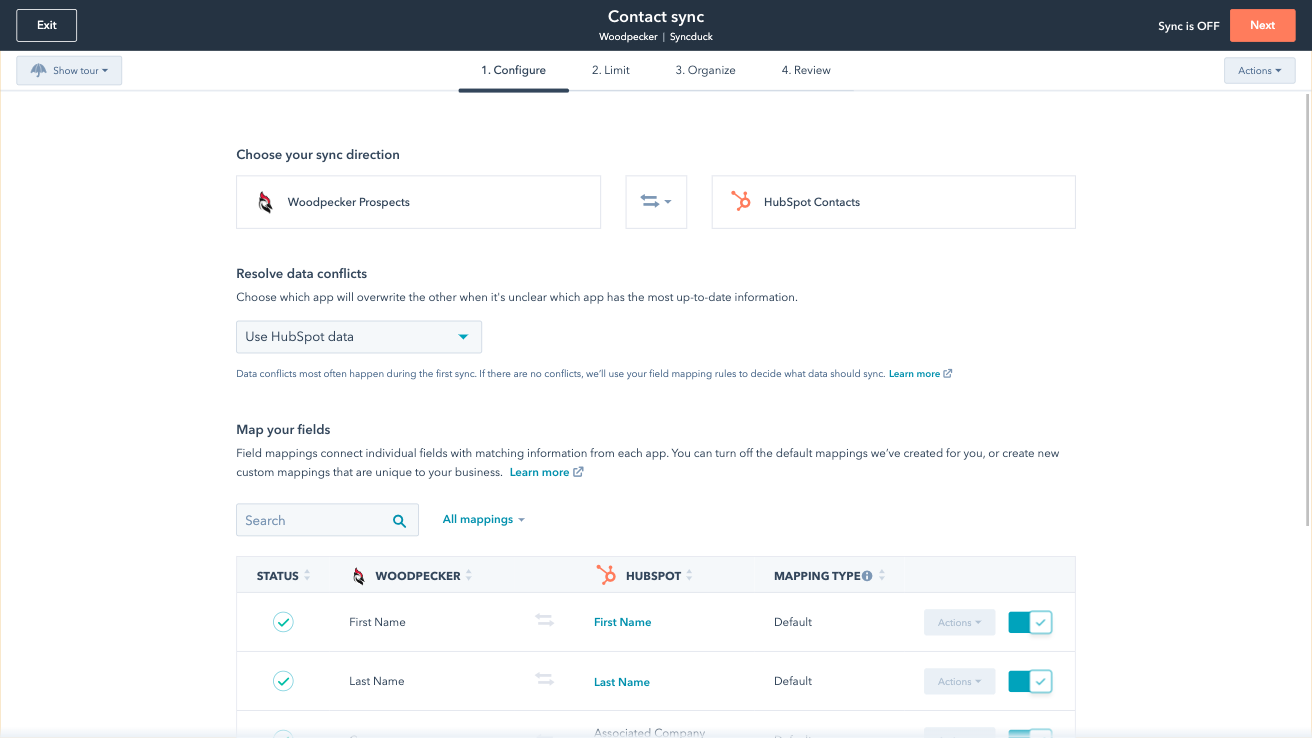**Detailed Caption:**

The image is a detailed screenshot of a software interface related to contact synchronization. The screenshot features a small font that's challenging to read without magnification. Upon closer inspection, the larger text reveals specific elements of the interface.

At the top, the headline reads "Contact Sync" with the subheading "Woodpecker/Syncduck (S-Y-N-C-D-U-C-K)". The synchronization setting is displayed to be "Off" in the upper right corner of the screen. Additionally, there are two prominent buttons: "Next" on the right side and "Exit" in the upper left corner. Accompanying these options is a "Show Tour" feature represented by an umbrella avatar.

Below the "Contact Sync" bar, there are four main sections: "Configure," "Limit," "Organize," and "Review." A directive prompts users to "Choose your sync direction" with options to synchronize between "Woodpecker prospects" and "HubSpot contacts," navigable via right and left arrows. The interface provides a solution for handling data conflicts, advising users to resolve discrepancies by choosing which application's data should take precedence, with a dropdown menu defaulting to "Use HubSpot data."

The screen also includes a section for "Map Your Fields." This function connects specific fields from each app, allowing users to turn off pre-set mappings or create customized mappings unique to their business requirements. Below this explanation, there's a "Learn More" link.

The interface features a search box for ease of navigation. At the bottom of the screenshot, a status line indicates the mapping between Woodpecker and HubSpot fields, with examples showing:
- First Name ↔ First Name (Default)
- Last Name ↔ Last Name (Default)

Overall, the screenshot serves as a guide for setting up and managing contact synchronization between Woodpecker and HubSpot, emphasizing configuration options and mapping details.